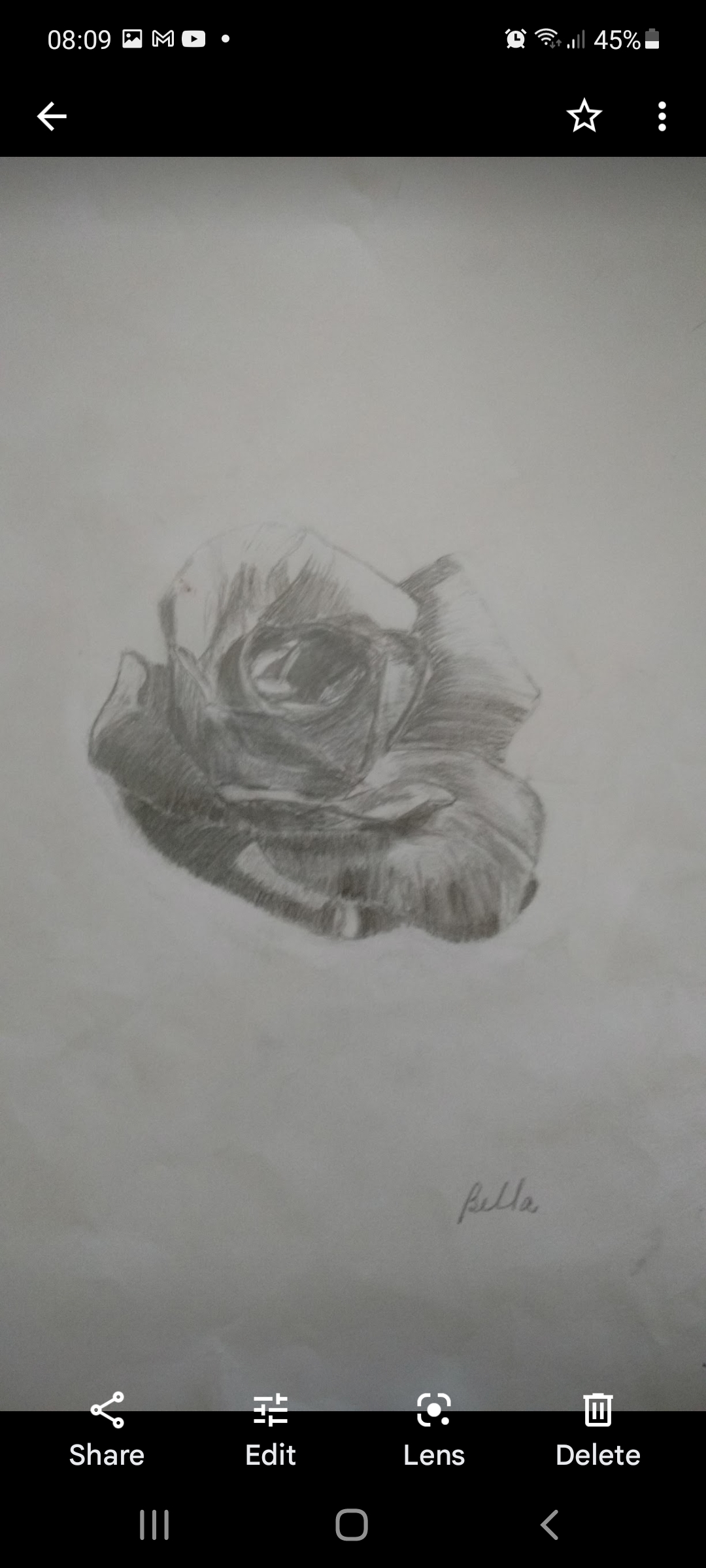The image is a screenshot taken from a smartphone showcasing a pencil drawing of a rose bloom. The sketch, which is done in shades of gray on white or off-white paper, features asymmetrical, curled petals that are more curved towards the upper left and larger towards the bottom right. Detailed shading gives depth to the flower, emphasizing its open, defined center. At the bottom right corner of the drawing, the artist's signature appears to be "Bella" in cursive. The screenshot captures typical smartphone screen elements: at the top shows the time, 8:09, battery level at 45%, and an active alarm. The bottom of the screen has icons for share, edit, lens, and delete, complete with their corresponding symbols. Below these icons, a thin black line appears, replicating the visual cue of a smartphone's navigation bar with three horizontal lines on the left, a hexagonal shape in the center, and an arrow pointing to the left on the right.